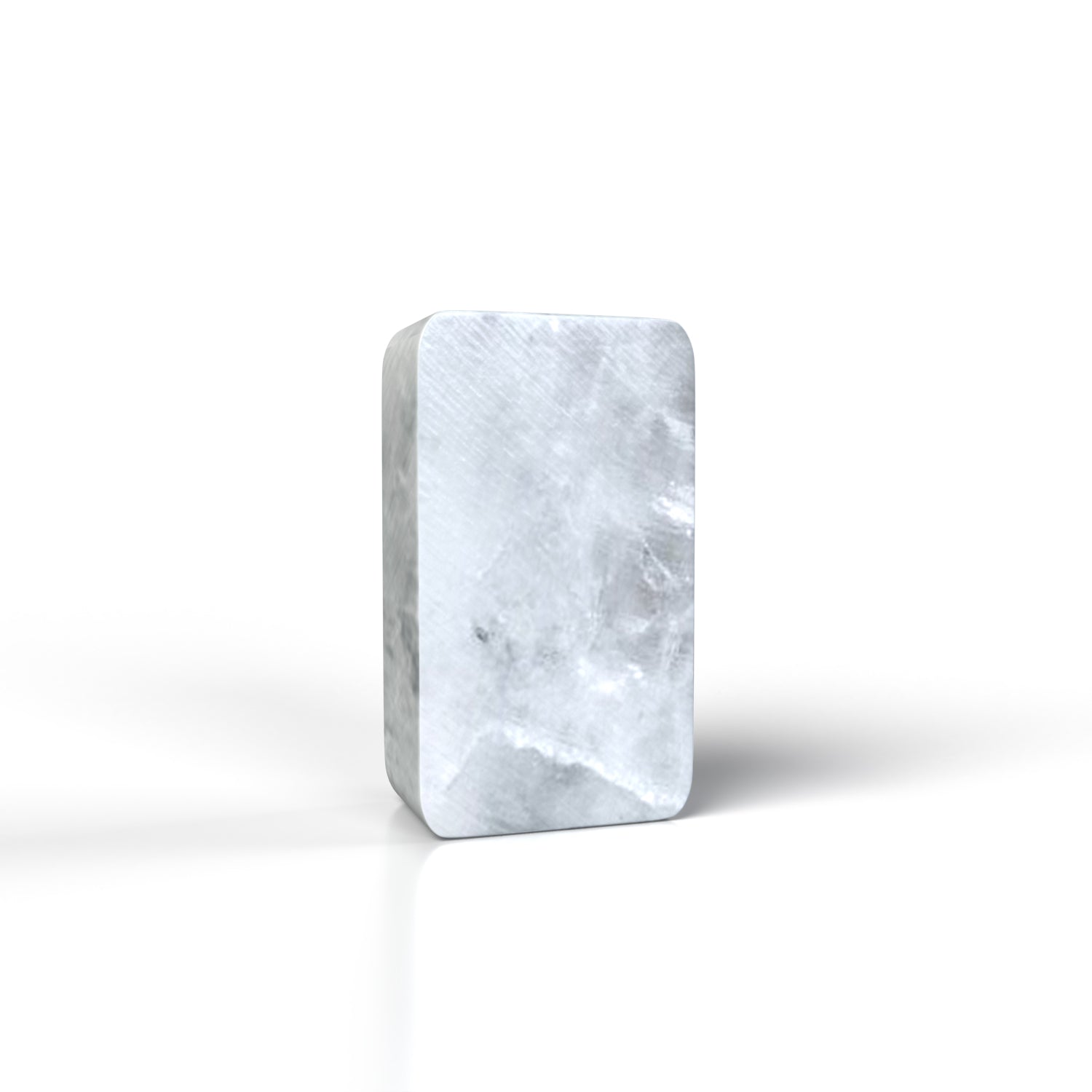The image features a thick, rectangular stone block with rounded corners, positioned at a slight angle on a white surface. The front and left sides of the block are visible, but its right side, top, and bottom are obscured. The top edge of the block is open, while the bottom edge rests firmly on the surface. Shadows cast by the block extend to the left, right, and rear but are absent in the front. The stone appears to be a type of marble or similar material, predominantly white with varying shades of gray. Gray areas interweave with intricate white lines or streaks, and a subtle saw kerf is visible, indicated by a series of fine circular lines etched into the surface.